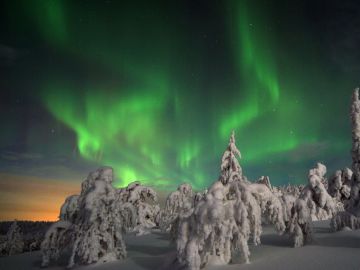This is a surreal nighttime photo set in a very cold environment. The ground and numerous trees, bent under the heavy weight, are blanketed in snow. In the background, a distant cliff edge is occupied by a series of statues that seem to be unearthly creatures, rendered indistinct by the perspective. Above, the sky is both alien and mesmerizing, dominated by wave-like, squiggly rays of green aurora borealis. The sky further features an orangish tint on one side, gradually darkening to a deeper gray above the horizon, enhancing the eerie and otherworldly atmosphere of the scene.